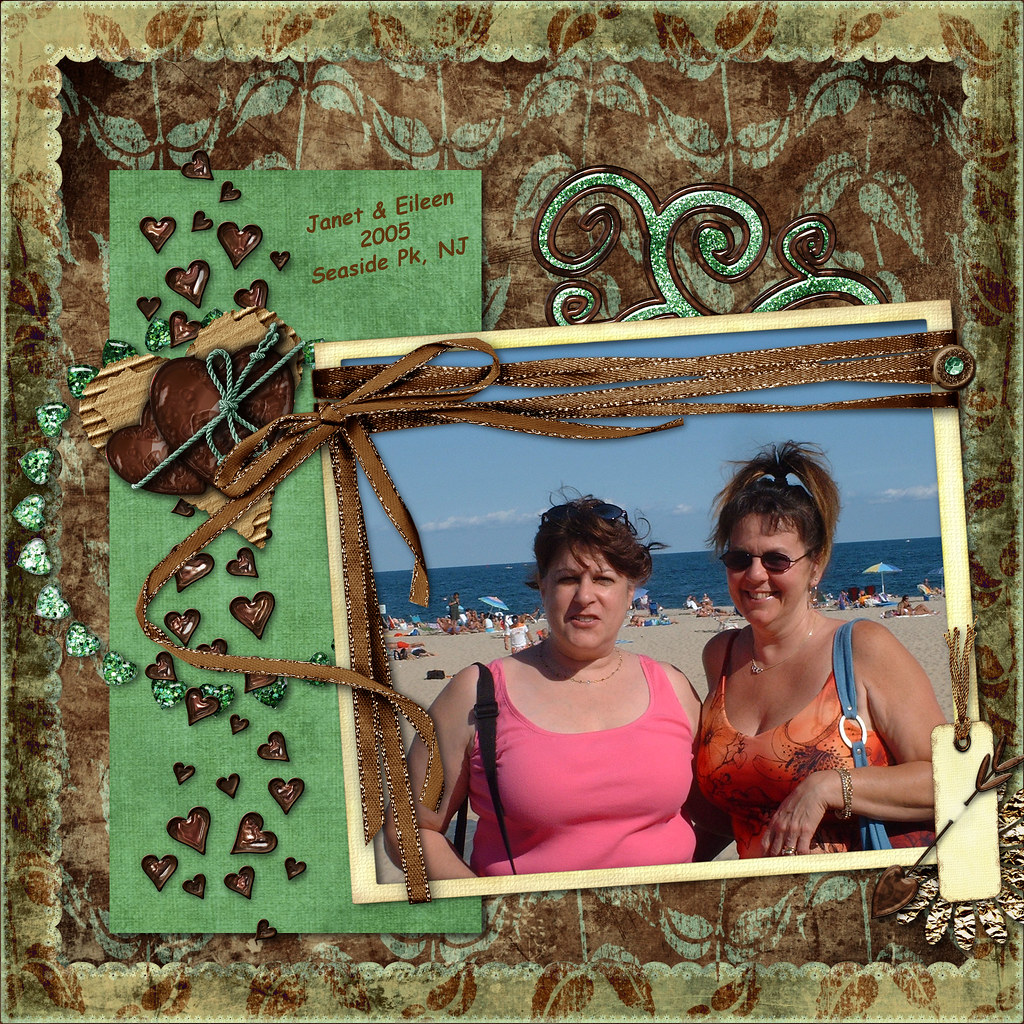This intricate digital photo collage mimics a scrapbooker's themed page and features a photograph of two women posing at Seaside Park, New Jersey in 2005. Set against a rich brown, gold, and slightly greenish floral backdrop with a metallic sheen, the collage includes a green card embellished with brown and teal heart-shaped jewels and cardboard cutouts, and inscribed with "Janet and Eileen, 2005, Seaside Park, New Jersey". The inset photo reveals a bustling beach scene with blue waters and either distant mountains or clouds on the horizon. Both women, Janet in a pink tank top with sunglasses perched on her head and Eileen in an orange floral tank top with sunglasses on, smile warmly at the camera. Each carries a purse, Janet's with a visible blue strap on her left shoulder. The photograph is bordered with a brown ribbon, adding to the scrapbook-like aesthetic.